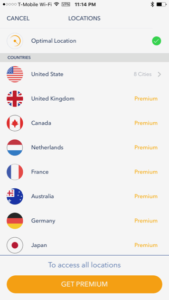The image displays a smartphone screen with detailed interface elements:

- At the top, the status bar indicates a weak T-Mobile signal on the left, followed by a Wi-Fi icon and text, the time (11:14 p.m.), an active Bluetooth icon, and a battery meter on the far right.
- Below the status bar, starting on the left, are multiple options such as "CANCEL" in all caps, "LOCATION," and various icons. Directly under the "CANCEL" button is an orange half-circle icon.
- The main content features a section labeled "ULTIMATE LOCATION" with a green checkmark on the right. This area is separated by a gray banner which displays "COUNTRIES" on the left.
- Below this banner, there are circular flags representing different countries, each with its corresponding name and status. For instance, the United States is marked with "8 cities," while other countries like the United Kingdom, Canada, Netherlands, France, Australia, Germany, and Japan are labeled "PREMIUM."
- A text in the middle of the screen explains that to access additional locations termed as "XL LOCATIONS," a PREMIUM upgrade is required.
- The background of the screen is primarily a light gray or off-white, while actionable items such as the green checkmark and PREMIUM upgrade option are highlighted in orange with white lettering.

The visual design aids in distinguishing between free and premium options, with the U.S. being the only free accessible location, whereas other countries require an additional fee.